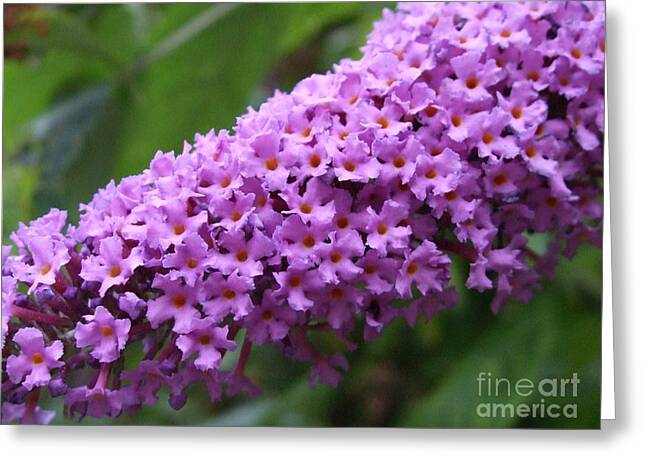This image depicts a graphic representation of a greeting card that's partially folded towards the viewer, revealing its white inside. The front cover of the card features a close-up photograph of purple flowers, likely lilacs or crocuses, displaying trumpet-shaped blooms in pinkish-purple hues with orange centers. These flowers are arranged in a conical stalk that extends diagonally from the bottom left to the top right of the image. The flowers stand out vividly against a blurred green leafy background, creating a striking contrast. In the lower right-hand corner of the card, there is an opaque white watermark that reads "Fine Art America" in lowercase sans serif font. The lighting suggests an overcast outdoor setting, and the overall presentation gives the card a 3D effect with shadows indicating the fold. This detailed and vibrant image would serve well as a sample for an online storefront, showcasing how this beautiful nature photograph could be printed on a greeting card.